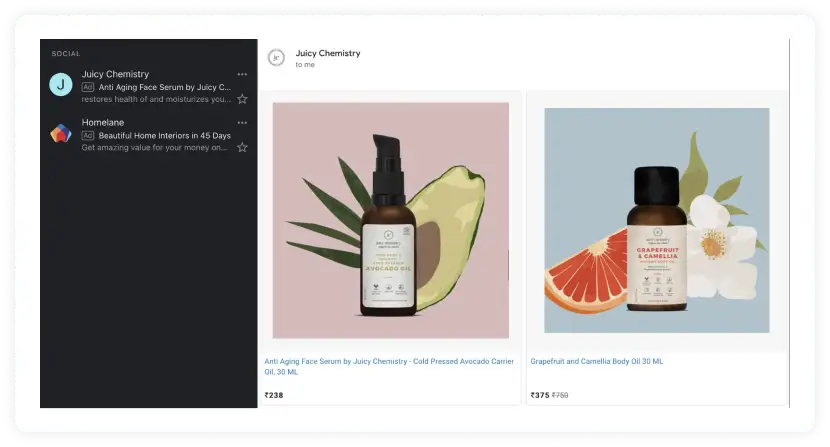**Caption:**

A screen capture of a website interface is prominently displayed. On the left side, there is a vertical black rectangle labeled "Social" in white lettering, indicating it is a section for social media comments. This section features two posts. The first post highlights "Juicy Chemistry" and specifies "Anti-aging Face Serum by Juicy C." Below, there is another comment about "HomeLane" with an advertisement for "Beautiful Home Interiors in 45 Days."

To the right, the content transitions to a product showcase. At the upper left of this section, it reads "Juicy Chemistry For Me." Below this heading are two images side by side. The left image features a bottle of serum with an artistic cucumber drawing in the background. The caption for this image reads, "Anti-aging Face Serum by Juicy Chemistry - Cold-Pressed Avocado Carrier Oil 30 ml." The right image displays another serum bottle against a background featuring a citrus wedge and a flower. The accompanying text for this photo states, "Grapefruit and Camellia Body Oil 30 ml."